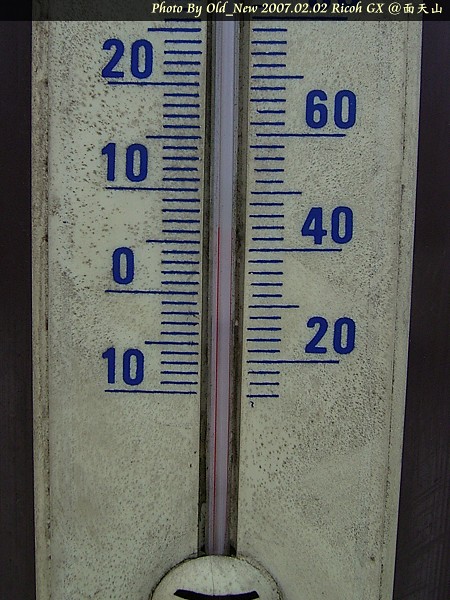The image features an old, weathered thermometer prominently displayed against a dark gray background. The thermometer's central position is flanked by narrow gray edges. The white plastic surface of the thermometer, eroded and pitted from prolonged exposure to the elements, exhibits numerous gray marks and pockets.

On the left side of the thermometer, numbers 10, 0, 10, and 20 are marked in blue, with additional blue lines indicating increments in between. On the right side, the numbers 20, 40, and 60 are displayed. A red line within the thermometer indicates a temperature reading of 43 degrees. 

At the very top of the image, the text "photo by old_new 2007.02.02 RICO GX" is visible, followed by three symbols that appear to be in an East Asian or Arabic script. The thermometer has clearly endured the test of time, as evidenced by its worn and weathered appearance.